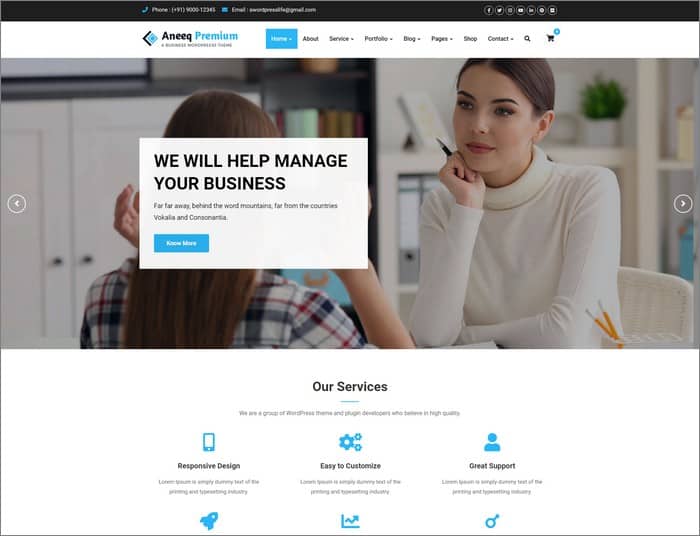On the Anik Premium website—spelled N-A-E-E-Q—there is a prominent feature image at the top of the page depicting a stock photo. In this image, a young female employee of the company is attentively listening to a potential client, who is also a young woman. The employee is dressed in a long-sleeved turtleneck sweater and holds a white pen or pencil in her right hand, indicating a professional and engaging atmosphere. 

Beneath the image, a text overlay reads, "We will help manage your business," accompanied by a call-to-action button labeled "Learn More." Scrolling further down, the site details the company's services, highlighting key features such as responsive designs, easy customization, and great support. Although the specific service offerings are detailed in small text, it is clear that Anik Premium specializes in WordPress themes and plugins that enhance website aesthetics and functionality. This website aims to provide tools that make your website appealing and highly efficient.